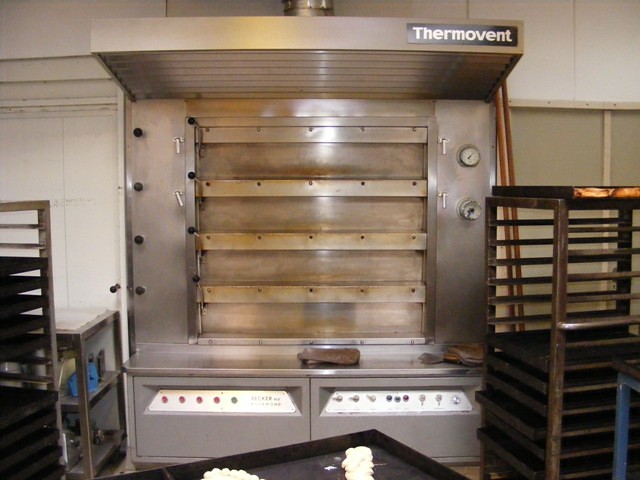This is a color photograph of an industrial Thermovent oven, likely used in a bakery or commercial kitchen setting. The machine has a distinctive stainless steel exterior with "Thermovent" inscribed at the top. The upper part features a prominent hood, enhancing its industrial appearance. Below the hood are four glass-covered sections with knobs along each side, indicating adjustable heating levels. In front of the oven, partially visible, is a black baking tray with two braided loaves of dough waiting to be baked. On both sides of the oven, tall baker's racks equipped with empty baking sheets provide ample space for holding trays of food, typical in a cafeteria or large kitchen. To the left, a silver kitchen prep table serves as a functional workspace, while the background showcases a white, industrial-looking wall, completing the professional kitchen setting.